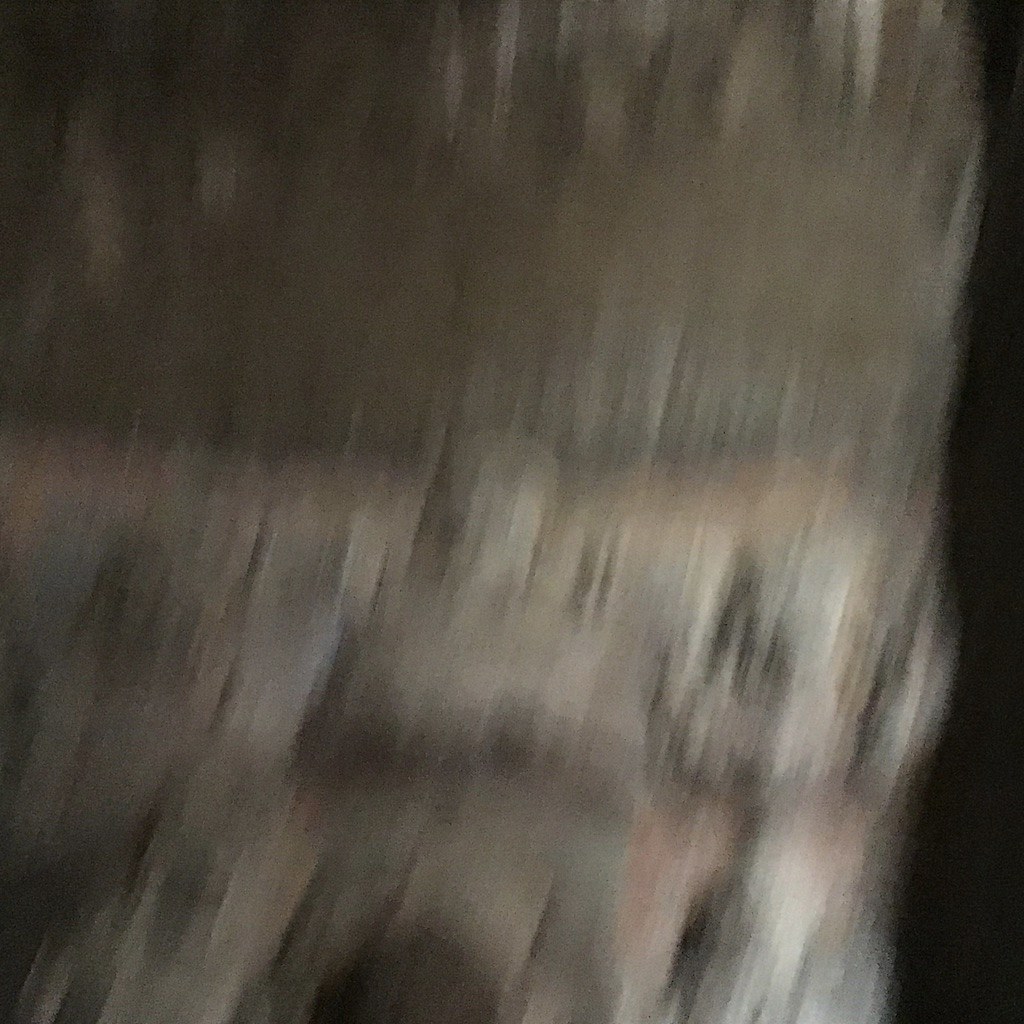The image appears to be taken inside a cavern or a similarly dark place, rendered extremely blurry as if the camera was moved quickly during the shot. The right-hand side fades into a strip of black, indicating deep shadow. The foreground shows a large, textured stone or rock feature, spanning from gray to hues of orange, red, and purple at the bottom. Despite the blur, the upper part of the image portrays more neutral tones of gray and brown. Centered within the composition, against what might be a stone wall, are the indistinct outlines of three figures: one central figure with hands clasped together, possibly in a seated position, and flanked by two others. The figure to the right seems to have arms outstretched, while the one on the left appears more humanoid or alien-like, making it ambiguous whether these are statues or actual human figures. This scene may depict an exhibit at a museum or a preserved historical monument, captured with very low quality and a great deal of motion blur.